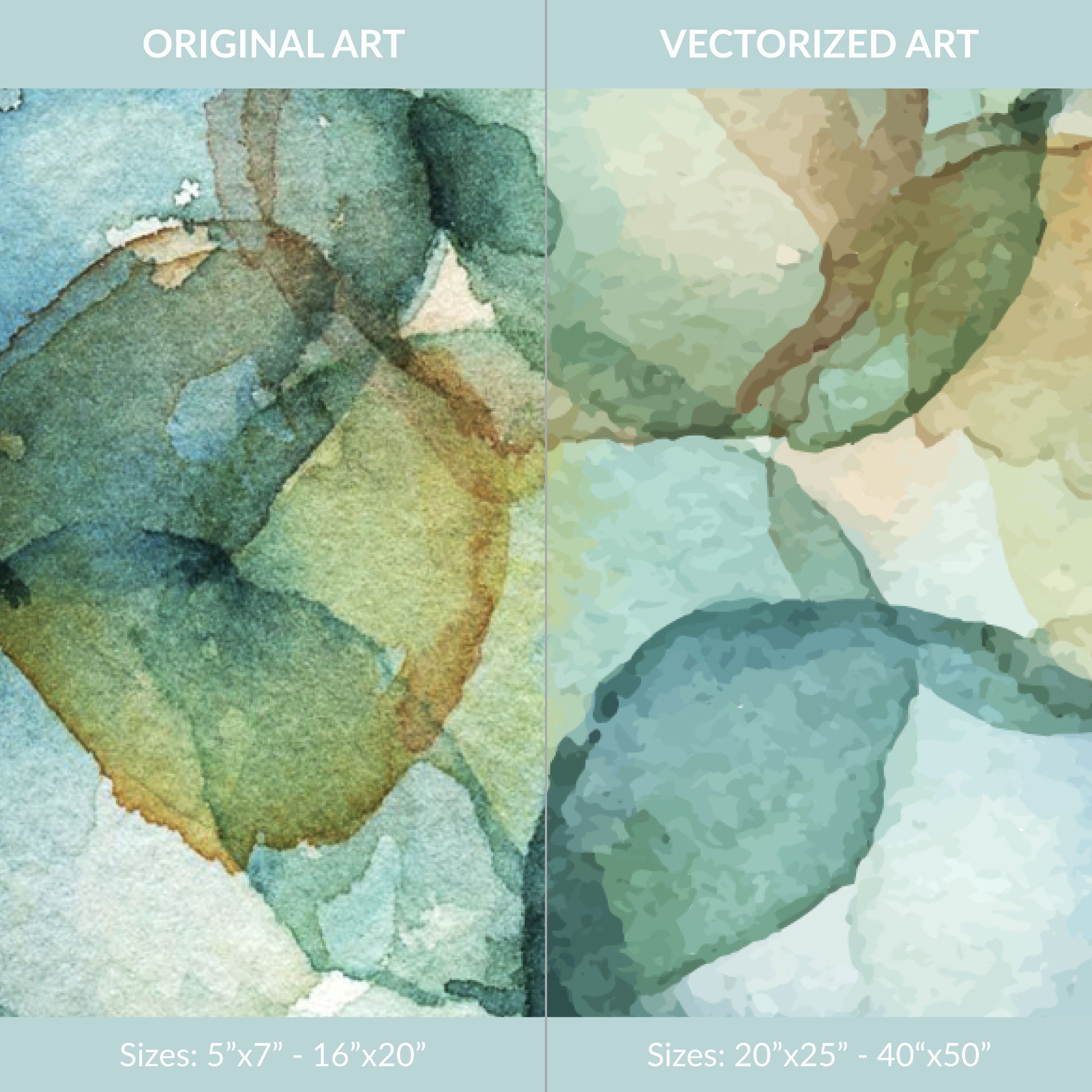The image displays two similar styles of abstract art side by side against a blue-green background. On the left, labeled "Original Art," it showcases a rough, watercolor-like painting composed of overlapping circles and edged squares, with blended shades of blue, green, yellow, and hints of brown and beige. This piece is available in sizes 5 by 7 and 16 by 20 inches. On the right, labeled "Vectorized Art," the same design appears but with a smoother, more polished look, almost resembling a glass texture. This version preserves the original's color palette but appears clearer and more refined, available in larger sizes of 20 by 25 and 40 by 50 inches. The two images align perfectly, forming a coherent, puzzle-like whole when viewed together.